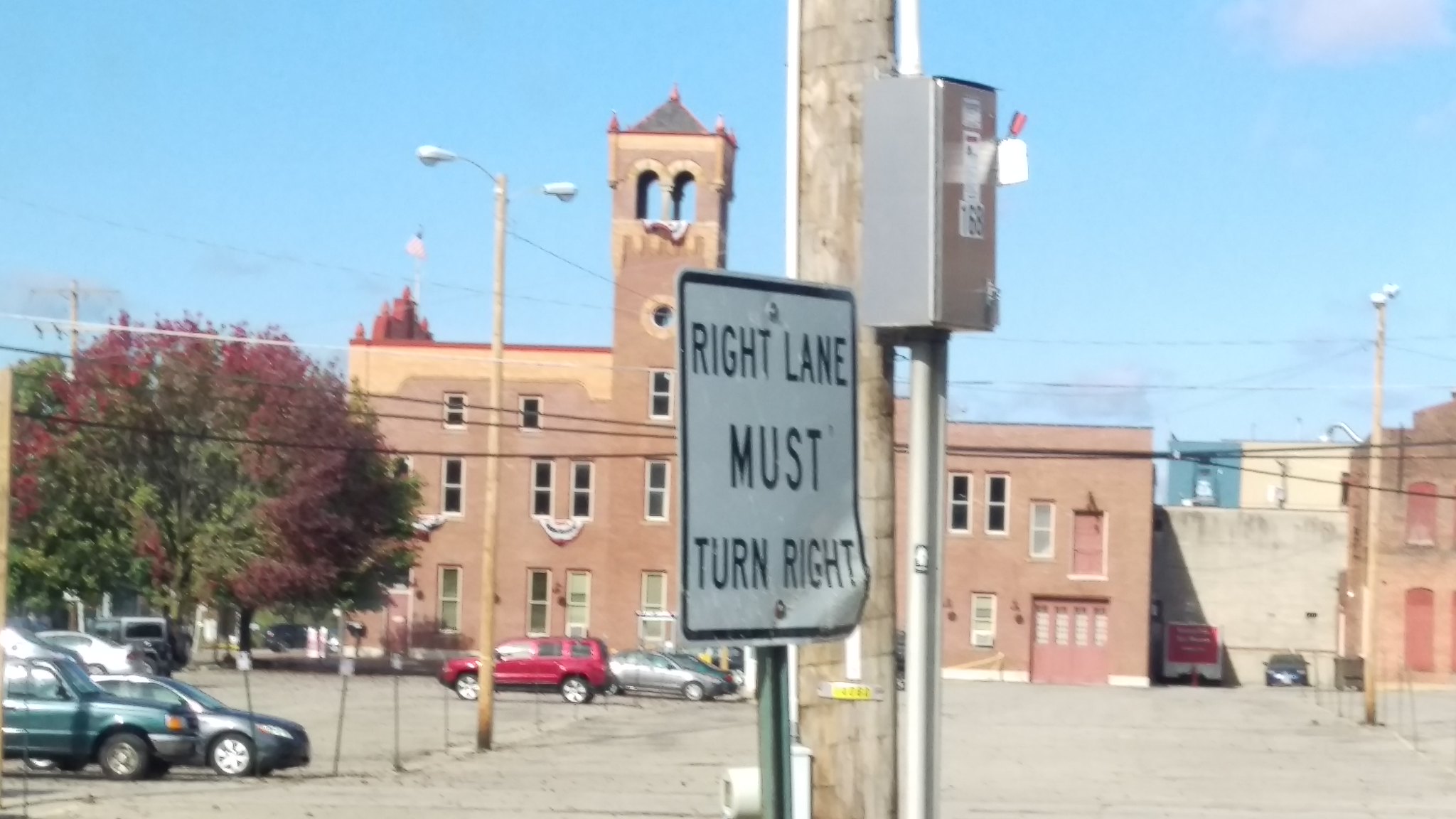In this detailed outdoor scene, a clear blue sky provides the backdrop for an expansive view of a town. Dominating the background is a grand red brick building featuring a tower adorned with a red, white, and blue banner near the top. The building's architecture includes a prominent round window and an array of rectangular windows across its three stories, suggesting it could be a historic or institutional structure, possibly a university or a church.

In the foreground, a slightly bent white sign with black lettering commands attention, stating "Right lane must turn right." This sign is fixed to a gray pole that ascends from the middle of the image. Adjacent to this is a larger brown utility pole, equipped with a silver metal box. 

To the left of these poles, a parking lot extends into the middle of the image, holding several vehicles: a silver car, a red SUV, a bluish-silver car, and a green SUV. An additional few cars can be glimpsed at the periphery. The image also captures various streetlights and telephone wires intersecting the scene. Additionally, on the far left, a tree with green and red leaves adds a touch of greenery beside another brown building. The overall composition paints a vivid and detailed picture of a bustling town environment, blending modern utilities with historic architecture.